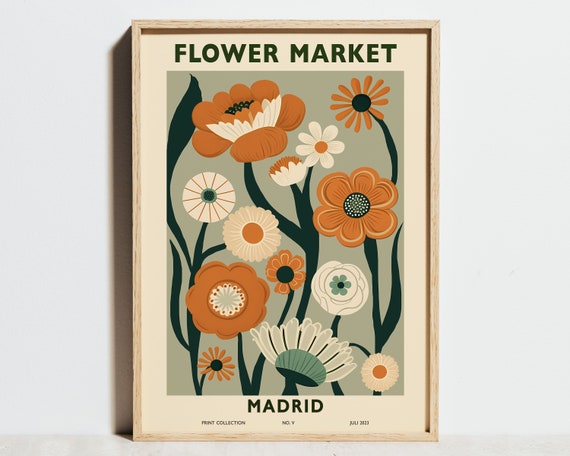This image captures a photograph of a framed drawing, seemingly a flyer, likely displayed at a flower market in Madrid. The frame, thin and wooden with a brown hue, encases an artfully illustrated collection of flowers. The top of the artwork prominently features the text "Flower Market" in green capital letters, while "Madrid" is inscribed at the bottom. In the lower corner of the frame, small text reads "print collection." The illustration itself is set against a serene, light blue backdrop and depicts a vibrant arrangement of florals. These flowers vary in shape and size, showcasing a mix of dark orange, white with orange centers, and rusty red petals, all connected by dark green or black stems and leaves. The color palette exudes a seventies vibe, with muted greens and creams blending harmoniously. The overall style of the drawing is cartoony, giving the piece a charming and whimsical aesthetic. The image suggests this framed artwork is propped against a wall, likely within the bustling environment of a flower market in Madrid.